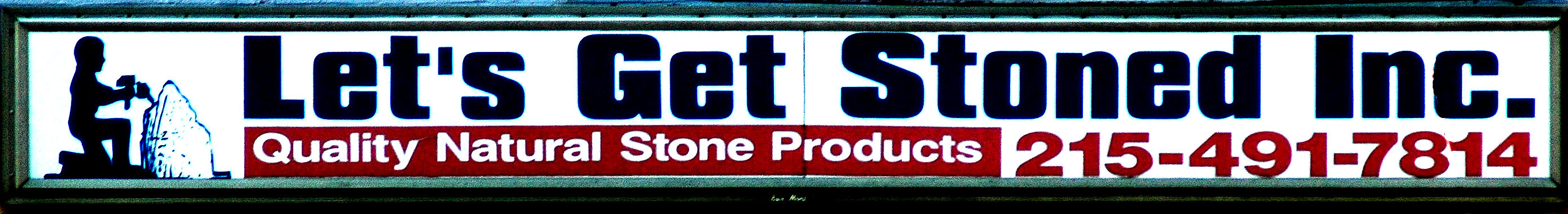The image showcases a small, horizontally narrow commercial sign bordered by a navy blue and light green frame. The main section of the sign is white and features black text at the top that reads, "Let's Get Stoned Inc." In the center-left of the sign, there is a dark blue silhouette of a kneeling man holding a tool, positioned in front of what appears to be a large white stone. Below the company name, there is a red rectangle containing the phrase "Quality Natural Stone Products" in white letters. Adjacent to this red box, the contact number "215-491-7814" is displayed in red text.